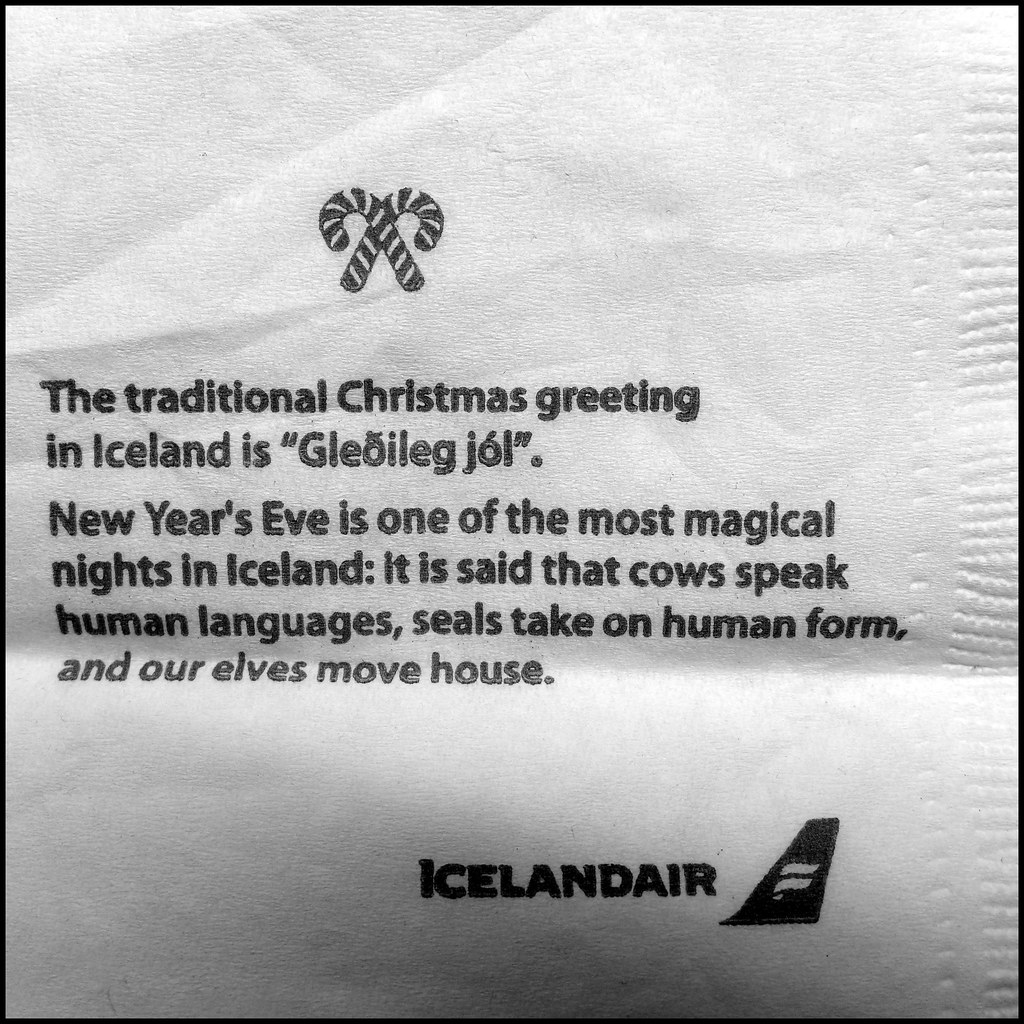The image is a close-up photograph of a textured, white napkin, prominently featuring multiple creases and folds. At the top center of the napkin, there are two black and white cartoon-style crisscrossing candy canes. In the middle of the napkin, the text in black print reads: "The traditional Christmas greeting in Iceland is Glóðeg jæsug. New Year's Eve is one of the most magical nights in Iceland. It is said that cows speak human languages, seals take on human form, and our elves move house." Below this, in the bottom right corner, the word "Icelandair" is printed alongside a logo resembling an airplane wing with a small white design on it. The image is rendered in shades of black, gray, and white, with the napkin taking up the entire frame, suggesting it might be from an Icelandair flight.